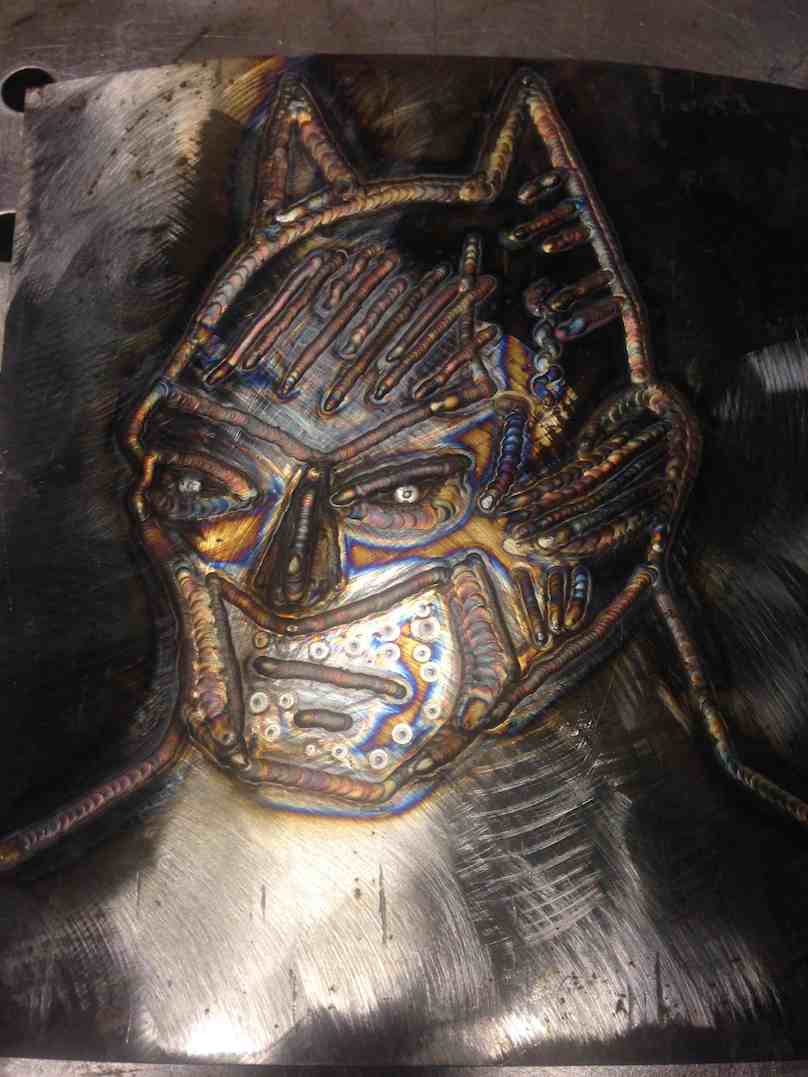This image showcases a detailed piece of artwork, seemingly created through welding on metal, featuring a Batman-like figure. The figure's mask has two pointed ears at the top, reminiscent of both a cat and Batman, earning it the nickname of "Batman Catman." The mask covers a cat-like body, with the face embellished with various colors and details. Around the mask's eyes, there are small, diamond-like elements, with hues of blue, orange, and green interspersed throughout. The top of the helmet is predominantly dark with vertical lines descending from the top. The face also features buttons and bejeweled sections in white and blue, giving it a structured and vivid appearance. The background appears to be a black or gray sheet of metal, adding to the artwork's industrial and artistic look.